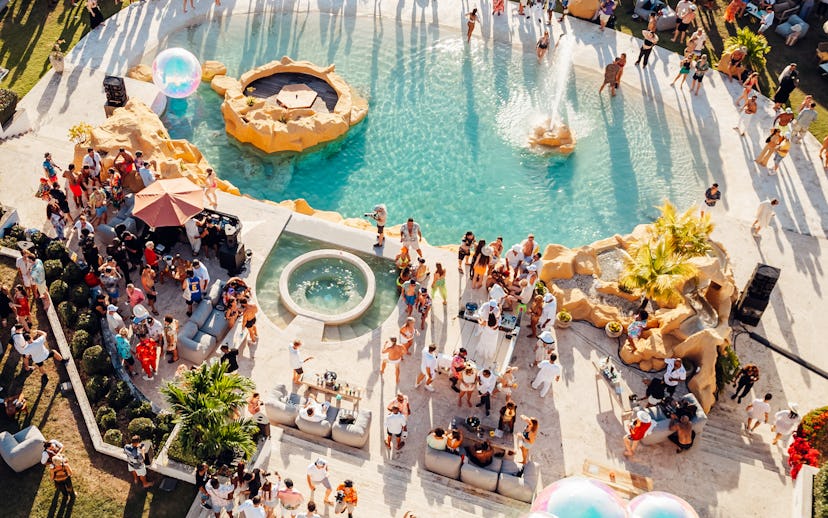An aerial photograph captures a lively pool party set around a stunning elliptical pool filled with vibrant blue water. At the center of the pool, a beautiful fountain surrounded by brown rocks adds an elegant touch. The ground surrounding the pool is a pristine white, and it's bustling with people enjoying the festivities, some lounging on single-seater sofas, others standing or walking. Shade tents and umbrellas provide respite from the sun, and lime green plants and trees add a touch of nature to the scene. There's a noticeable spa or hot tub area adjacent to the pool and steps on the right where people can be seen ascending and descending. The atmosphere is relaxed and cheerful, with party-goers in summery white outfits, adding to the uplifting vibe. Beyond the white ground area, a lush grassy expanse extends, dotted with more people enjoying the event. A giant beach ball floating around adds a playful element to this vivid summer gathering.